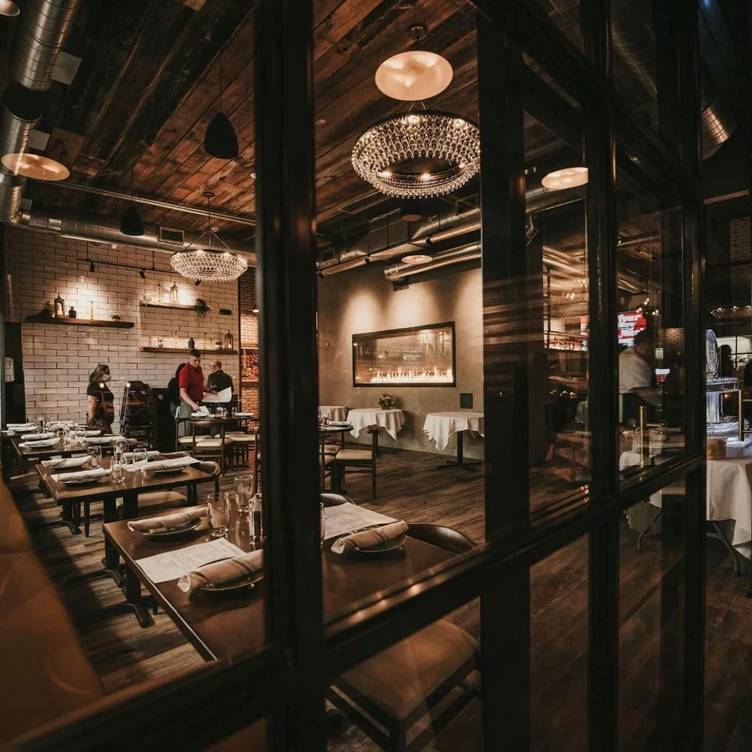This dimly lit, upscale restaurant features a striking interior with dark wooden flooring and a matching ceiling made of brown cork wood. Two elegant, round crystal chandeliers hang from the ceiling, casting a soft glow over the space. The walls are adorned with a gray brick pattern, enhancing the sophisticated ambiance.

Guests are seated at rectangular, heavy wooden tables, set with plates, silverware, and folded napkins. Some tables are covered with white tablecloths, and centerpiece caddies hold various seasonings. On the left side, booth-style seating with brown upholstery adds a cozy touch to the establishment.

Towards the back of the room, a large screen is mounted on the wall, and three people are visible. A man in a red shirt, possibly a musician, stands with what seems to be a guitar strapped to his back. He is accompanied by a woman in an apron, possibly a staff member overseeing the setup. Another man in a black shirt appears to be assisting them. The scene is framed by large windows, giving a glimpse into the bustling and refined atmosphere within.